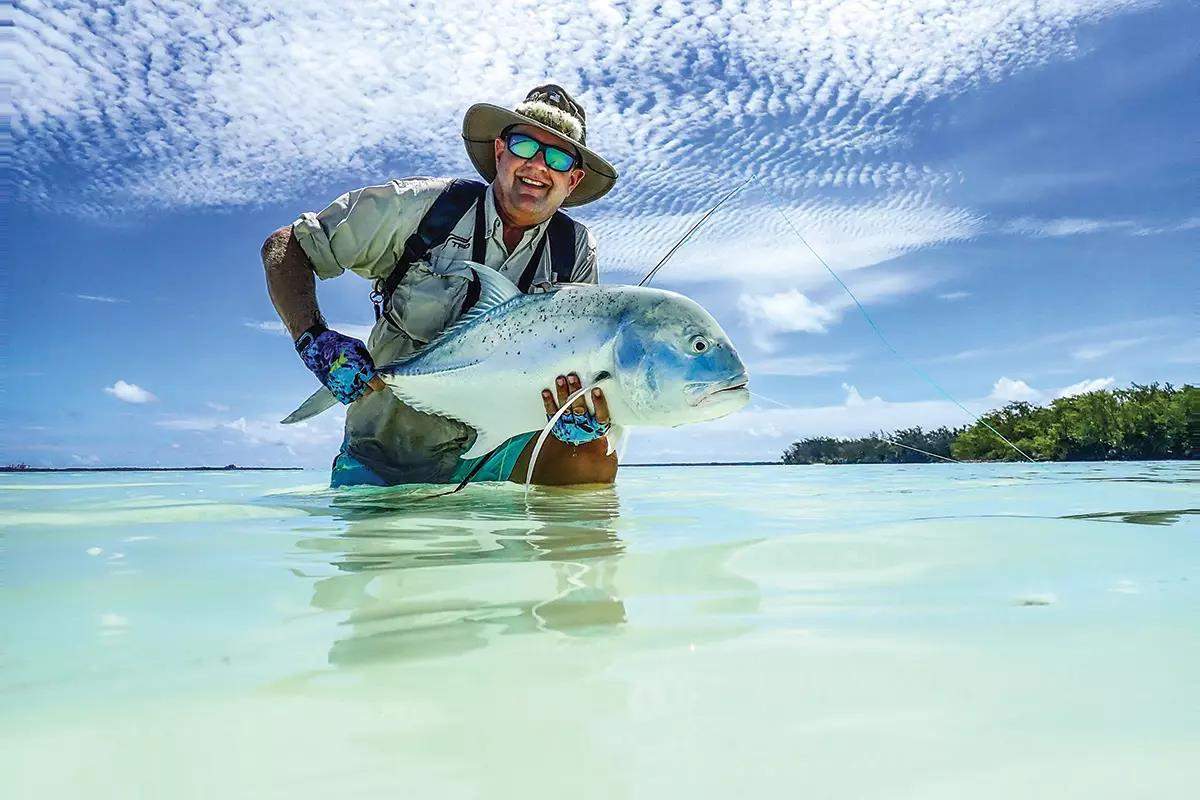The photograph captures a smiling fisherman kneeling in crystal clear, knee-deep water in a tropical setting, holding a sizable blue fish. His attire includes a floppy brimmed hat, polarized reflective sunglasses, and a khaki shirt with sleeves rolled up to the elbows, revealing blue fingerless gloves. The fisherman also wears a backpack with visible black straps. The fish he cradles, characterized by its wide face, open eye, and slightly gaping mouth, exhibits a gradient from blue at the top to white at the bottom, and has prominent fins on its back and stomach. The serene background features a bright, sunny blue sky with sparse, choppy clouds and an island with visible trees on the right side of the horizon. The water, light blue and crystal clear, allows the sandy bottom to be seen easily, enhancing the tranquil ambiance of the scene.